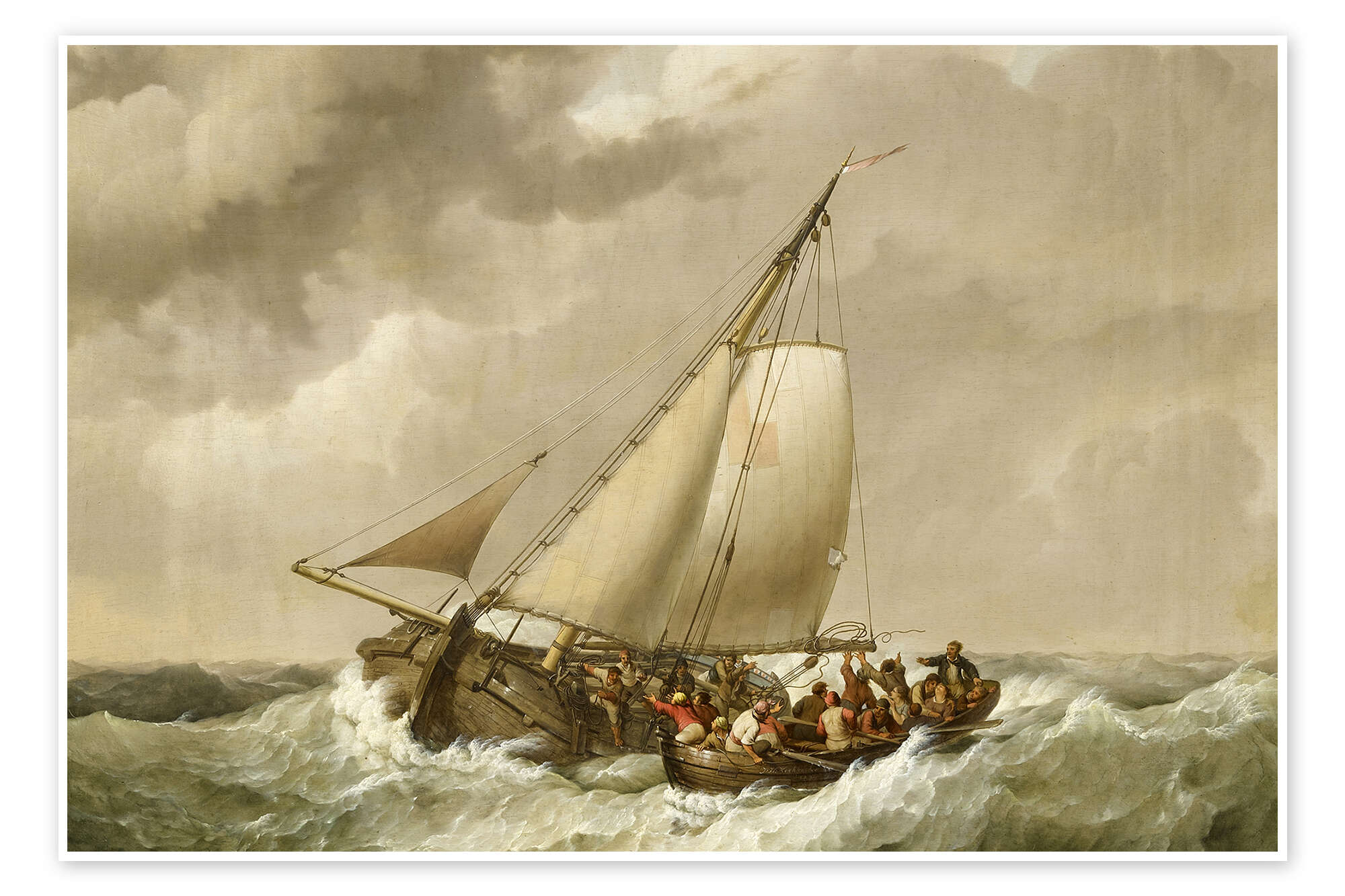The painting depicts an intense and dramatic scene of a shipwreck caused by a violent storm in the ocean, with immense, towering waves crashing against an old-fashioned schooner. The vessel, equipped with three sails and intricate rigging, appears to be on the verge of sinking amidst the tumultuous, grey seas. The atmosphere is dominated by dark, rain-filled clouds casting a bleak, monochromatic tone over the entire scene, except for the vivid red jackets worn by some of the men, which starkly stand out. 

The composition captures a desperate rescue operation: some men are already precariously seated in a brown wooden rowboat, while others, clad in white and khaki clothing, are either reaching out for help from the lifeboat or attempting to climb aboard from the main ship. This action-packed image illustrates the peril and urgency faced by the sailors. 

The overall muted palette and style suggest the painting might originate from the 1800s, evoking a sense of historical seafaring adventure and tragedy. The painting is presented with a white border, indicating it is a print likely sold online.